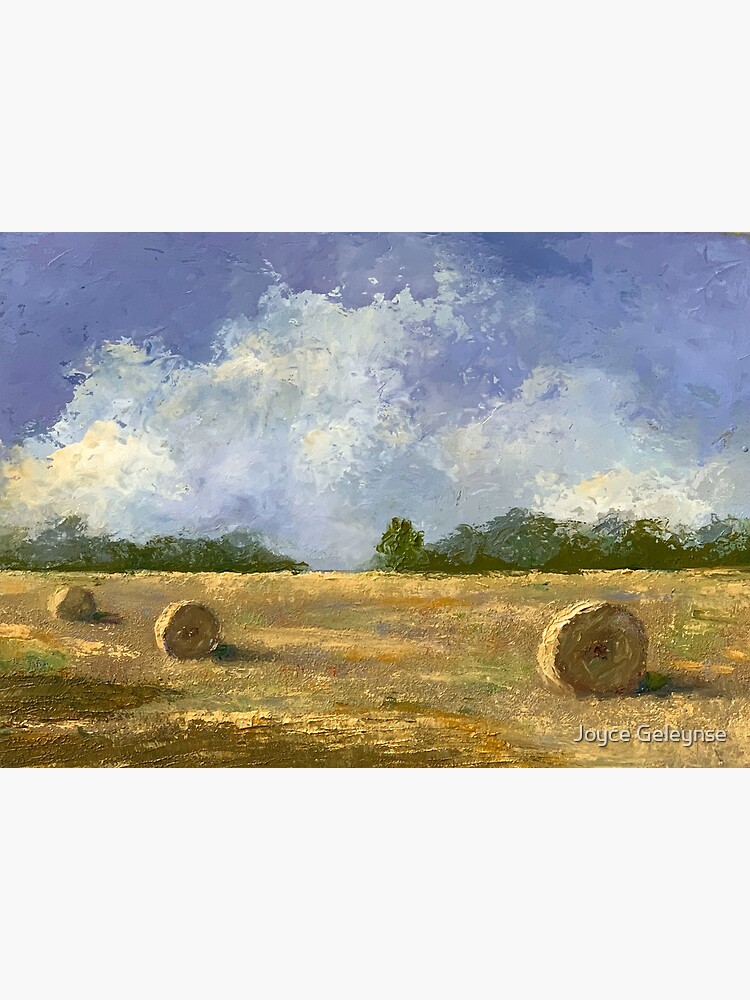This is a detailed painting of a farmland scene, prominently featuring a vast beige field that appears texturally rich due to visible paint strokes. The field showcases three large cylindrical hay bales with holes in the middle, arranged in descending size from right to left, set against golden and dark brown hues interspersed with patches of green. The painting transitions at its middle into a horizon adorned with lush green bushes and trees, above which fluffy white clouds float in a serene blue sky. It's notable that the painting is wider than it is tall, adding to the expansive feel of the landscape. The lower right corner of the artwork bears a watermark signed "Joyce Geleynse" in white, set against a black background. The painting itself is mounted on a white wall, enhancing its natural tones and inviting closer examination of its textural details.